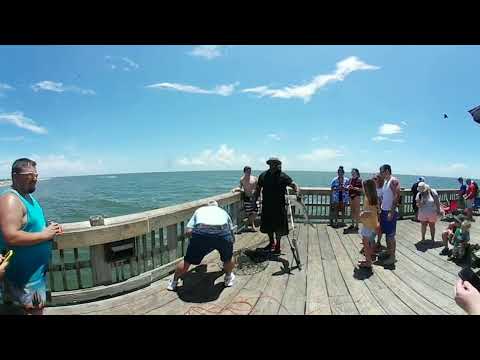The image depicts a bustling wooden pier extending into a calm ocean, with serene greenish water and blue skies adorned with several white clouds. The pier is bordered by wooden railings, giving a quaint charm to the setting. A diverse crowd of men, women, and children are engaged in various activities along the pier, dressed in casual summer clothing. Prominently, two people on the left side are involved in fishing, with a man bending over, seemingly trying to catch something, while another, a black male holding what looks like a small shark, captures the attention of onlookers. The scene is lively with approximately 20 people, including a shirtless man in swim trunks and a child accompanied by a kneeling woman. A man in the front of the scene, wearing a blue tank top and cactus-patterned shorts, stands holding an object in his hand, his short brown hair and glasses giving him a distinctive look. Everyone appears to be absorbed in the sunny, peaceful environment of the pier, where a shared sense of curiosity and leisure permeates the air.